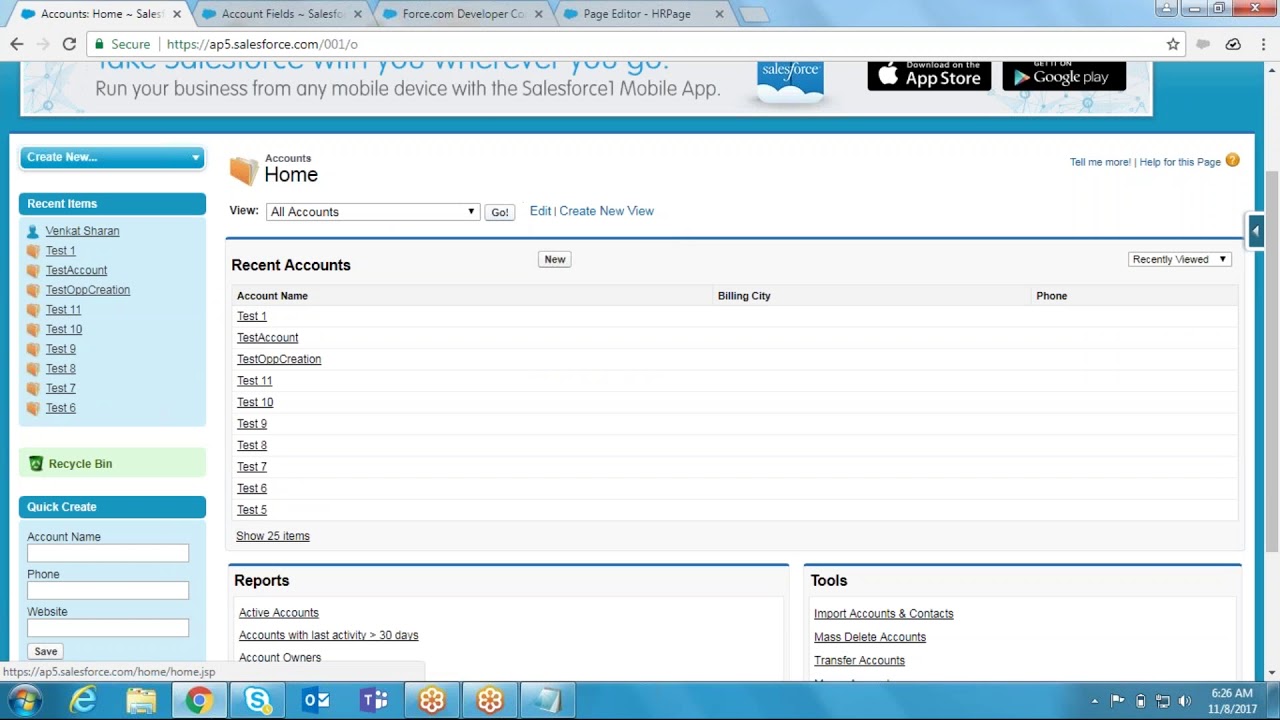The image displays a web browser with four tabs open. The active tab is labeled "Accounts Home," and the URL in the address bar reads "ap5.salesforce.com/001/0." Scrolling down shows the "Account Home" page, with a sidebar on the left featuring navigation options such as "Recent Items." The "Recent Accounts" section is expanded, listing various accounts in a left-justified format: Test 1, Test Account, Test Op, Creation, Test 11, Test 1, Test 10, Test 9, Test 8, Test 7, Test 6, and Test 5.

A dark blue teal-colored line separates this list from a section titled "Reports," which provides links such as "Active Accounts," "Accounts with Last Activity Less Than 30 Days," and "Account Owners." Further options seem to be available but are not fully visible. On the right side of the screen, there is a "Tools" section that includes options like "Important Accounts and Contacts," "Mass Delete Accounts," and "Transfer Accounts." The overall layout appears to be a typical account management interface in Salesforce.